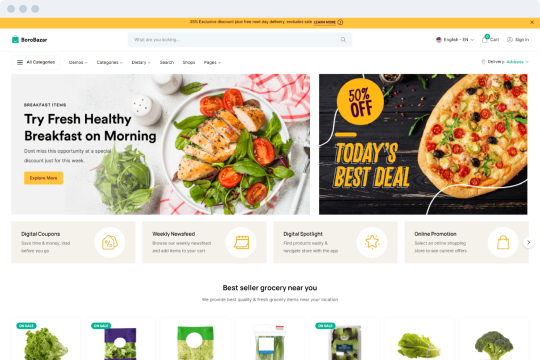Here is a revised and detailed caption for the described image:

---

The image is a detailed mock-up of a website, featuring a light bluish off-white browser window at the top with three grayed-out dots positioned on the upper left. Just beneath this browser window, there is an orange banner with completely illegible black text. 

Following the banner, the primary background color of the webpage is white. The visible logo, although unreadable, includes a distinctive green bag icon accompanied by black text. Adjacent to the logo, there is a search text input box, and nearby are several clickable elements, one of which resembles a cart icon with a green indicator. However, the number inside the cart is indistinct.

Further down, there is a horizontally scrollable section consisting of promotional images. The first visible promotion encourages users to "Try Fresh Healthy Breakfast in the Morning" and showcases an appetizing salad with grilled chicken, tomatoes, and a small bowl of herbs. To the right of this section, there is another promotion featuring an oval-shaped vegetable pizza topped with olives and tomatoes. It highlights a deal in yellow text that reads "Today's Best Deal" with a circular label indicating "50% Off."

Below these promotions, there are four clickable boxes offering various coupons. Underneath this section, there is a heading that reads "Bestseller Grocery Near You," followed by a row of seven visually appealing promo shots of different vegetables.

---

This caption should provide a clear and organized description of the website mock-up image.